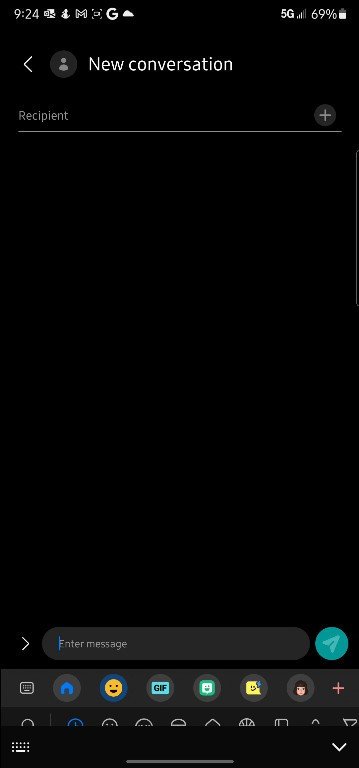The image depicts a smartphone screen displaying a new text message window against a black background. At the top of the screen, white notification symbols and text indicate the time as 9:24. Additional icons include a mail notification, a workout symbol, a Gmail notification, a Google logo, and a weather symbol on the top-left corner. The top-right corner shows the phone's connectivity status, including a 5G signal indicator with three out of five bars and a battery level at 69%. Below these notifications, there is a white back arrow next to a gray user icon and the text "New Conversation" in white. Underneath, there is a recipient field with a box featuring a plus symbol on the right side for adding contacts to the conversation. Following that, a large black box occupies most of the screen space, possibly for message display or input. At the bottom, another gray box labeled "Enter message" is present, accompanied by icons for emojis, GIFs, and the keyboard.